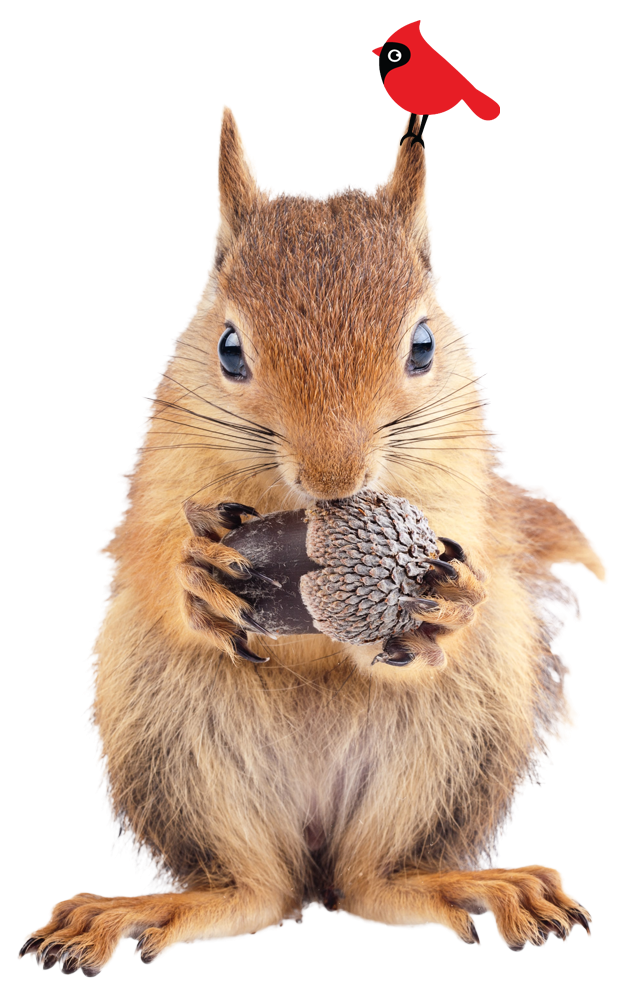This highly detailed close-up image features a realistic-looking squirrel clutching a brown acorn tightly with its sharp, uncut claws. The squirrel's mouth is in contact with the head of the acorn, which is held sideways between its paws. Positioned on a white, transparent background, the squirrel’s tannish fur with brown and black accents stands out prominently, and its large black whiskers are clearly visible. Its feet are planted firmly on the "invisible" ground in a V-shape. The squirrel is facing directly at the camera with both eyes fixated straight ahead. Adding a whimsical touch, a small, cartoonish red cardinal with an orange beak and black facial markings perches atop the squirrel's right ear (the left ear from the squirrel's perspective).